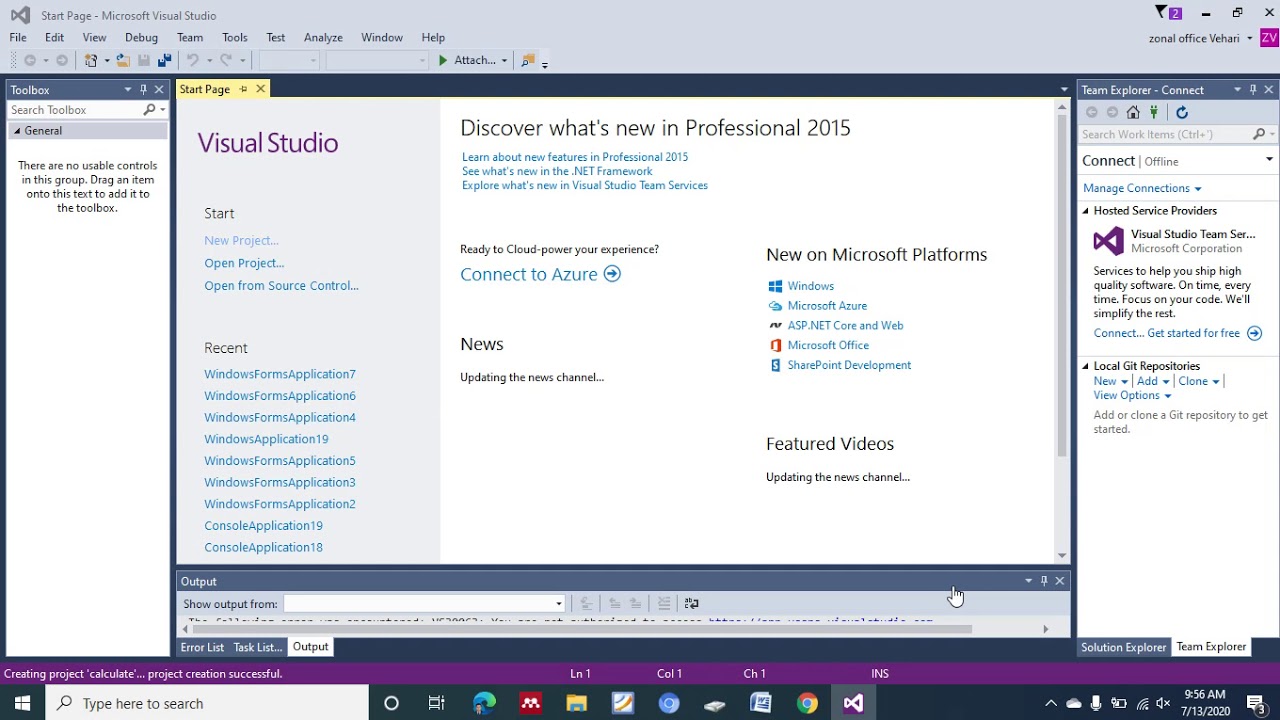A screenshot of the Microsoft Visual Studio desktop application is displayed, presenting a comprehensive view of its start page interface. At the top, a gray title bar appears with several control icons on the right, including a flag, a purple question mark, and buttons to minimize, maximize, or close the window. Below the title bar is a horizontal menu list featuring options like File, Edit, View, Debug, Team, Tools, Test, Analyze, Window, and Help. 

On the right-hand side of the bar, an integration label titled "Something Office" is shown, followed by a stylized logo containing the initials "ZW" or "ZV" enclosed within a box.

Beneath the menu bar, a left-aligned panel titled "Toolbox" includes a search function labeled "Search Toolbox General" and a message that reads, "There are no usable controls in this group. Drag an item into this text to add it to the toolbox."

Dominating the center of the screen is the Visual Studio logo, prominently featured in purple. Beside it, the text "Discover What's New in Professional 2015" opens introductions to new features, updates in the .NET Framework, and advancements in Visual Studio Team Services. Below these introductory statements are actionable options, such as "Start New Project," "Open Project," and "Open from Source Control." Under these choices, a list of recently accessed projects, including "Windows Forms Application 7" and others, is presented for quick access.